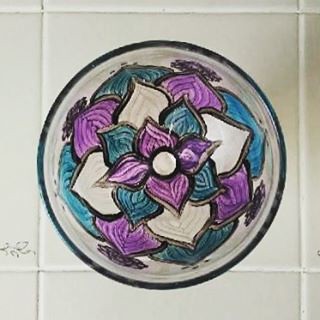In this detailed image, we observe a glossy white ceramic tile, which could potentially be part of a bathroom wall, kitchen backsplash, or floor. Central to the tile is a circular adornment, giving the impression of a sun catcher. This round image appears to be glass and seamlessly blends with the tile, making it difficult to discern whether it is an integral part of the tile or an addition affixed to it. The focal point within the circle is a three-dimensional flower design showcasing vibrant purple petals, accented with green and white leaves. The intricate floral motif stands out against the plain white backdrop of the tile, creating an eye-catching decorative element. No text is present in the image.